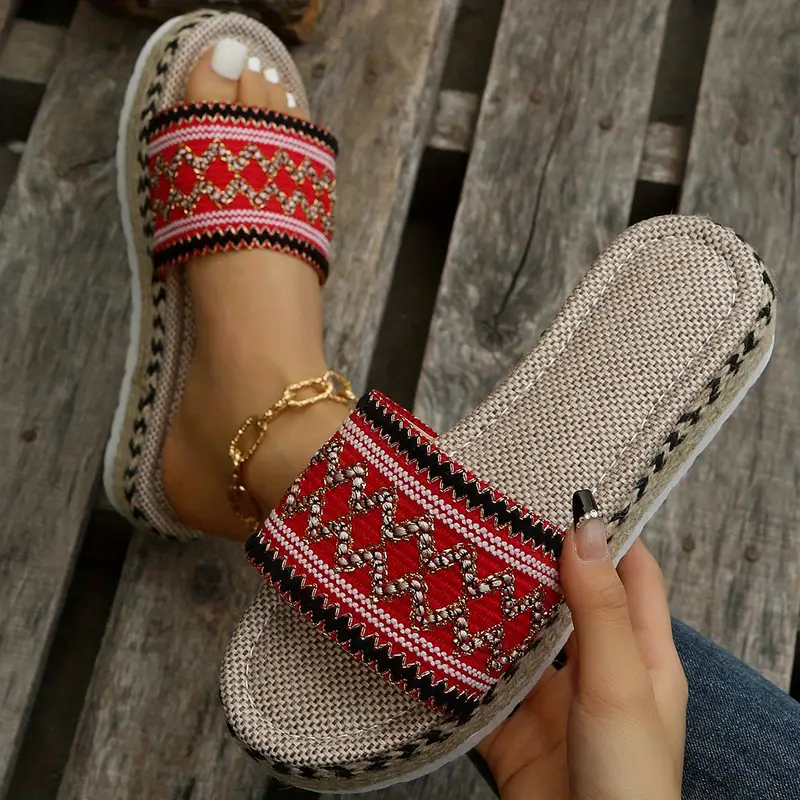The photograph captures a detailed scene of a woman with elegant features and accessories. She is sitting with her feet resting on a weathered gray wooden pallet, composed of widely spaced, distressed boards. The woman showcases her right foot adorned with a chic, flat, slip-on sandal. This sandal features a cushy white sole and a burlap-like footbed, outlined intricately with a rope design. A broad red strap with black zigzag appliqué and white rickrack patterns, forming diamond shapes, secures the sandal to her slim, pretty foot. Her toenails are meticulously pedicured and painted white, and her ankle is graced with a thick gold chain anklet. Meanwhile, her left sandal is held toward the camera in her hand, displaying her long fingernails with black tips and embellishments on an otherwise unpainted nail. The photograph also reveals that she is dressed in dark denim, adding a casual yet sophisticated touch to the overall composition.